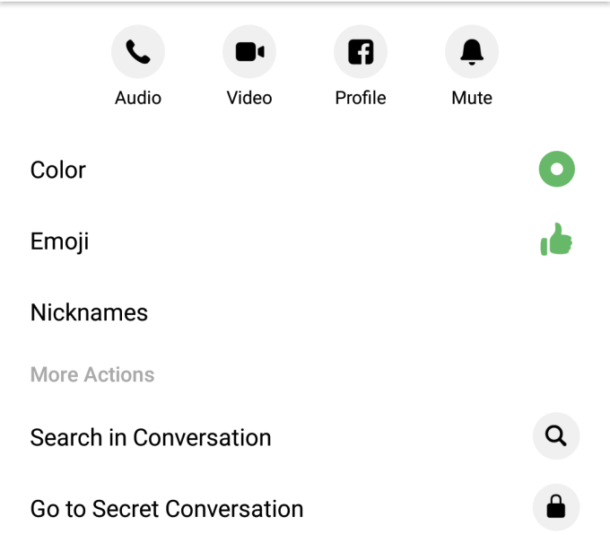This screenshot captures the settings interface of an app on a smartphone, featuring a clean light gray bar at the top. Directly beneath this bar are three evenly spaced light gray circles, each iconized and labeled: a phone icon with "Audio," a camera icon with "Video," a Facebook icon with "Profile," and an alarm bell icon with "Mute." 

In the main section under these icons, six options are listed vertically along the left side of the screen: "Color," "Emoji," "Nicknames," "More Actions," "Search in Conversation," and "Go to Secret Conversation." Opposite "Go to Secret Conversation," a small gray circle features a lock icon, symbolizing security. Above that, next to "Search in Conversation," is another small circle, housing a search icon, facilitating easy navigation within conversations. The layout is intuitively designed to streamline user interaction and settings customization.